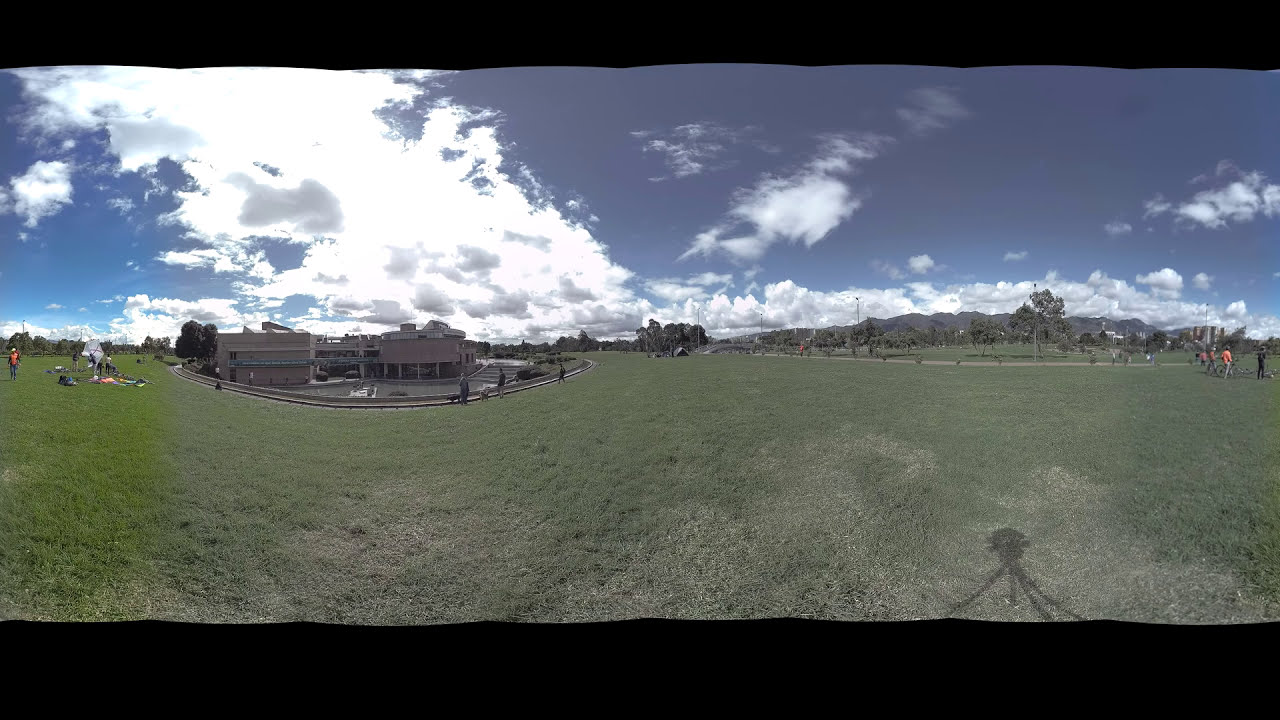This panorama view showcases a sprawling grassy field, stretching from the left to the right of the image. On the far left, a group of people is picnicking, lounging on blankets, and standing, creating a social atmosphere. Just beyond them, a small parking lot and a long brick building are nestled in a slightly depressed area, giving an interesting layering to the landscape. In the center left, the field continues with a few more people standing with dogs near the edge of the grass.

The right side of the image features expanses of greener grass, blending into areas of bluer-gray grass, with scattered individuals walking and one person pushing a bicycle. Much of the right is open field with a walking path visible near the foreground. In the background, a distant road runs parallel to the horizon and mountains rise above it.

Above this serene scene, the upper half of the photograph is dominated by a deep blue sky, adorned with patches of bright white clouds. A notable formation of clouds extends from the center of the picture towards the left in an upward diagonal. This daytime outdoor scene is encapsulated within a black header and footer, with the footer being thicker, framing the tranquil panoramic view.